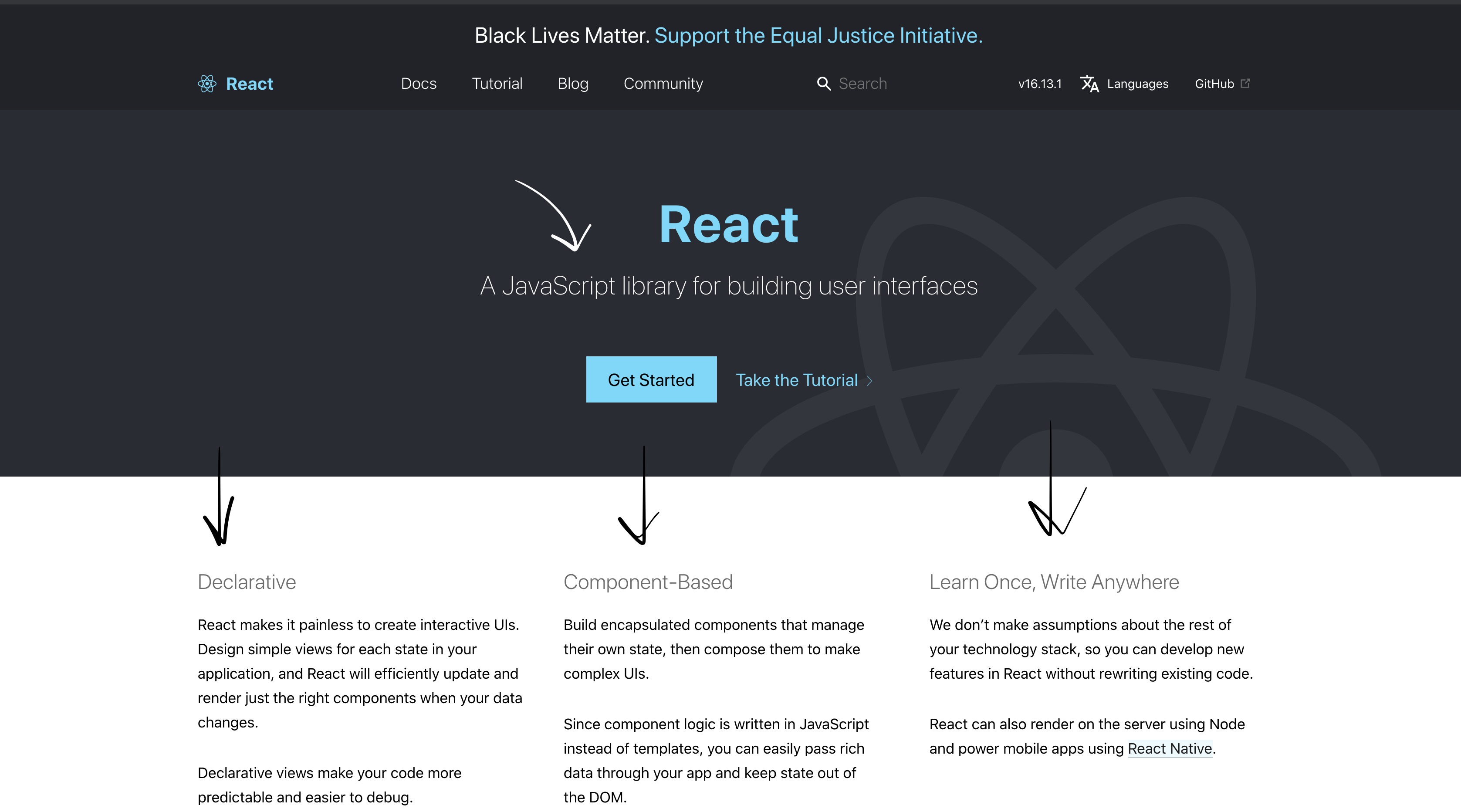This image showcases a Black Lives Matter website page with a sleek, dark black banner at the top. Centrally positioned on the banner is the phrase "Black Lives Matter" followed by "Support the Equal Justice Initiative," highlighted in an aqua blue font reminiscent of the color of the sky. 

On the left side of the page, there is an icon resembling a nucleus, paired with the bold, sky blue word "React." Adjacent to this, to the right, are navigational links labeled "Docs," "Tutorial," "Blog," and "Community." Also on the right side, there's a magnifying glass symbolizing a search function, accompanied by the word "Search," although the actual search box is not visible. Below this, language options are listed under the label "Languages."

Centered below, the title "React" is displayed in a large, sky blue, bold font. An arrow beneath it points to the description, "A JavaScript library for building user interfaces." Further down, there is a sky blue rectangular button labeled "Get Started" and another link "Take the Tutorial," marked with an arrow pointing to the right.

Three distinctive downward arrows guide the viewer towards sections titled "Declarative," "Component-based," and "Learn Once, Write Anywhere," each followed by descriptive paragraphs. At the bottom of the page, "React Native" appears to be highlighted, although visibility is slightly unclear.